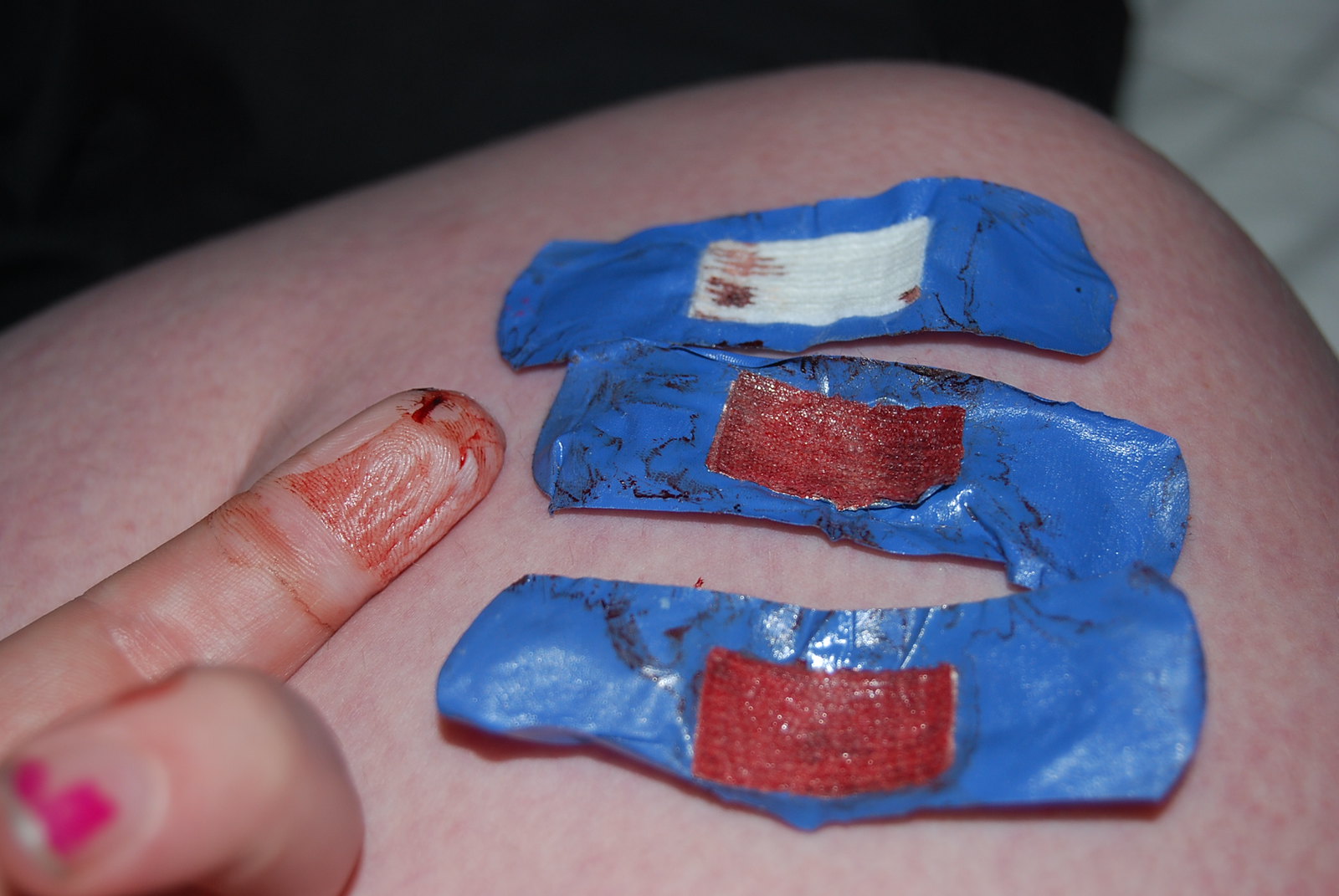In this color photograph, we see a detailed and somewhat graphic close-up of someone's injury and its aftermath. The primary focus is on a right leg, which appears to be bent at the knee, possibly crossed over the other leg. Lying across the knee are three blue band-aids, each with a white gauze pad in the center. All three band-aids are visibly stained with blood, with the middle one completely soaked, spilling onto the blue adhesive parts.

To the left, prominently featured, is a right hand with the palm facing up. The index finger has a small, bloody cut near the left upper corner, showing signs of having been freshly unwrapped from bandages; you can see an imprint where the band-aid had been. The finger's skin appears wrinkled and pruned, indicative of prolonged exposure to moisture. Adjacent to this finger, the middle finger is bent over, adorned with chipped pink nail polish.

In the background, the upper part of the image hints at a black object and a small patch of white that might be a corner of a bedsheet, further adding context to the scene. The overall impression is a raw snapshot of someone's attempt to tend to a minor injury, complete with the aftermath of used band-aids and a visibly bloodied finger.